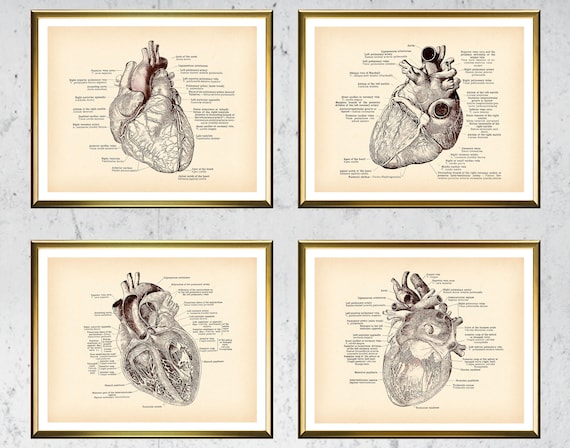This image showcases a wall adorned with four intricately framed medical illustrations of the human heart. Each illustration is meticulously presented in a thin gold frame with a white matte background and set against a gray, marbled wall. The drawings, done on an oldish beige paper, display the heart from various anatomical perspectives, each annotated with detailed lines and text that invite closer examination, though the print is too small to be legible in this depiction.

The top left illustration centers on a frontal view of the heart, highlighting the arteries extending from the top. Adjacent to it, the top right illustration offers a top-down perspective, revealing the complex network of veins and arteries, alongside prominent ventricles. The bottom left image presents a cross-sectional view, exposing the interior chambers of the heart, cut in half to reveal the structure within. Finally, the bottom right illustration provides yet another unique angle, emphasizing the top and one side of the heart, completing this comprehensive visual study of the organ's anatomy.